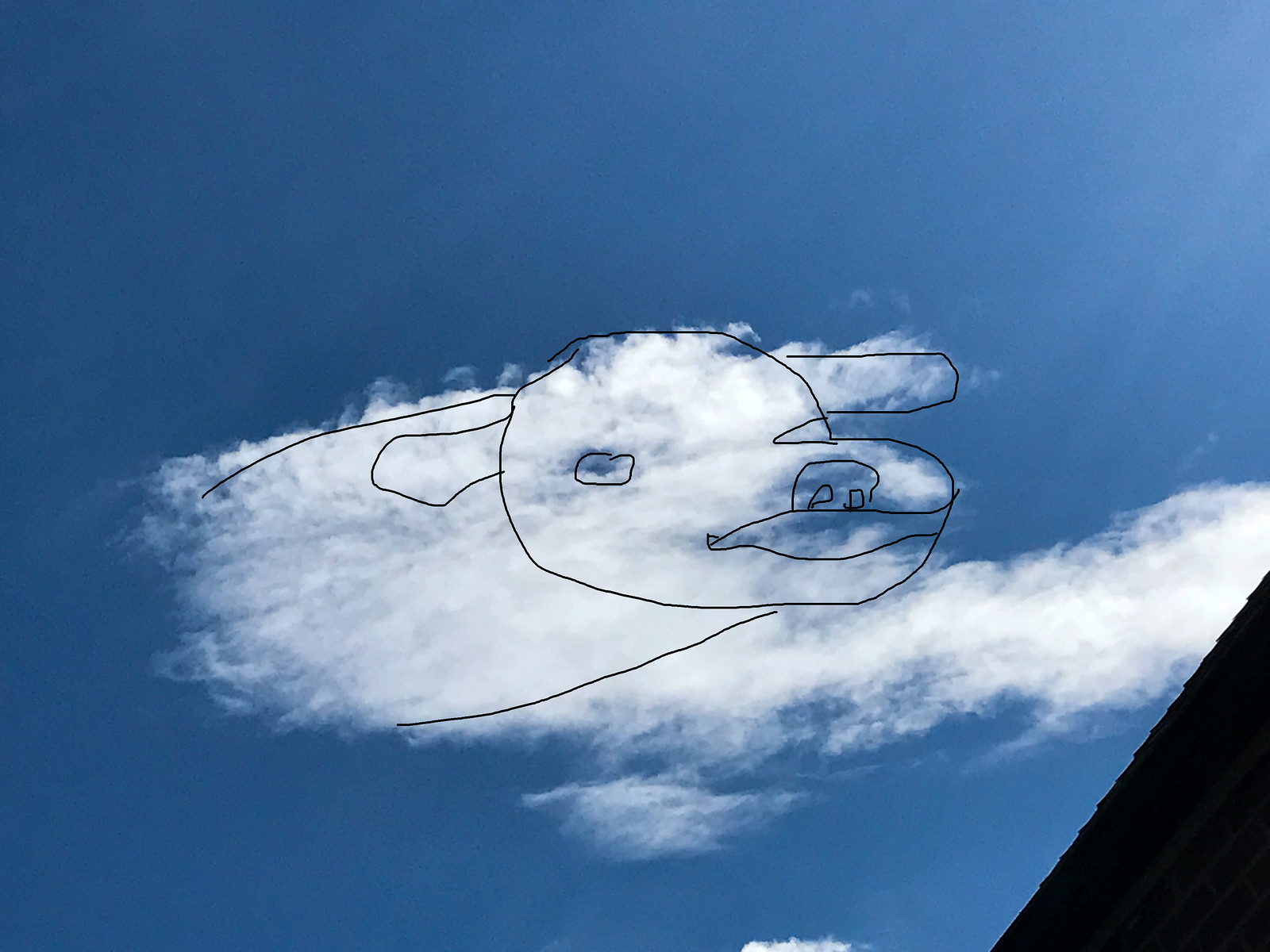This color photograph features a vibrant blue sky dominating the scene, with a large, white, fluffy cloud almost centered but extending towards the right-hand edge. The cloud takes up about half of the photo's height and three-quarters of its width. In the lower right corner, there's a dark, serrated-edge triangle, likely the roof of a house with tiles.

At the heart of the cloud, there's a whimsical line drawing overlay. It depicts an animal’s side profile, which could be interpreted as either a pig, dog, or cow, based on its features. The drawing showcases two oblong ears protruding from the top of the head, a rounded snout with a nose, an open mouth, and one circled eye. The animal’s body is suggested by an incomplete oval shape, with the cloud's border serving as part of this outline. No limbs are visible in the drawing. The overall effect is an amusing melding of natural cloud shapes with playful human artistry.